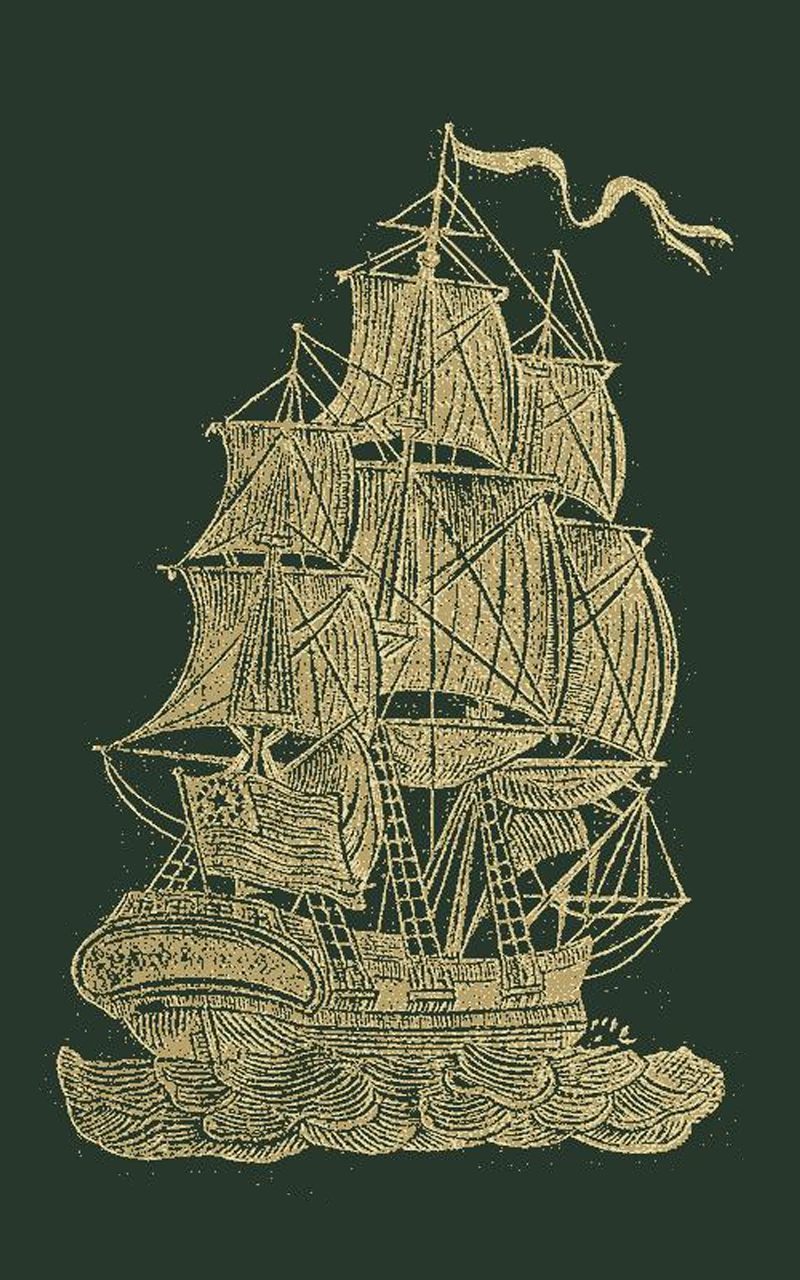The image is a detailed print of a large, yellow-tinted sailboat set against a dark green background. The overall shape of the image is rectangular, with the left and right sides being twice as long as the top and bottom sides. The depiction shows the ship from the back and side, highlighting multiple levels of sails, each grouping featuring three sails. The ship's intricate design outlines are rendered in a sandy, beige color, giving it a grainy texture reminiscent of sand art. Waves, formed by gold lines, add to the dynamic sense of motion. An American flag, with its stripes and stars on a small square at the corner, is positioned at the stern of the ship, while a skinny flag flies from the very top. The scene evokes a sense of historical or possibly Norse maritime adventure.